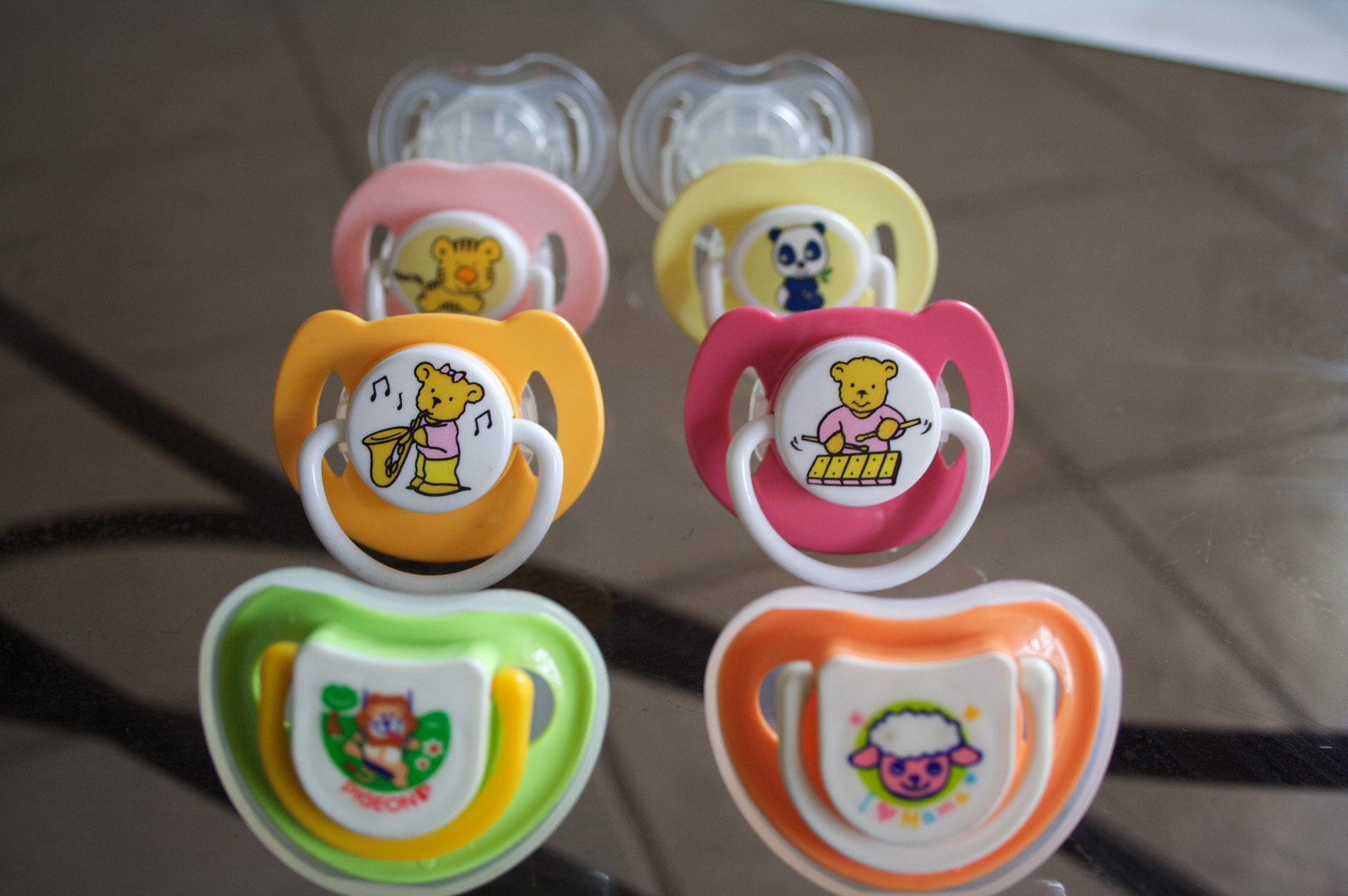This photograph captures eight baby pacifiers neatly arranged in two rows of four, placed on a glass table. The background features a slightly out-of-focus brown tiled floor. Each pacifier is of a different color and design. Starting from the back row, the two pacifiers on the far left are clear plastic with no designs. The pacifier to their right is peach-colored with a cute yellow tiger featuring an orange nose on a white circular front. To its immediate right is a pale yellow pacifier adorned with a small panda bear.

Moving to the front row, the first pacifier on the left is a yellow-orange color displaying a bear playing a saxophone. This bear is dressed in a pink shirt and orange-yellow pants, complete with a bow on its head. Next to it is a deep pink pacifier featuring another bear playing the xylophone, wearing a pale pink shirt. The third pacifier on the left in this row is slightly out of focus but appears lime green with a design of an indistinct animal in a meadow. Lastly, the bright orange pacifier on the far right has a pink lamb with white fluff on its head.

Each pacifier's vibrant colors and adorable animal designs make them stand out, despite the varying focus. The glass table and tile background add a clean, organized look to the composition.